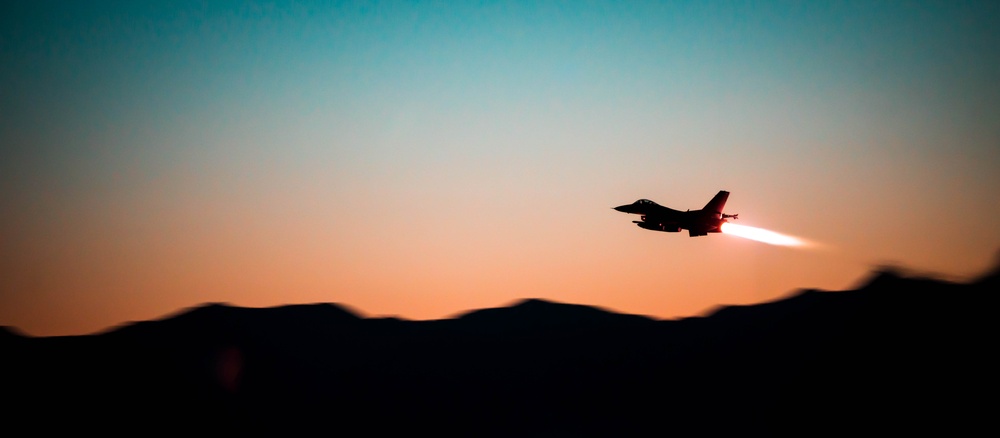This photograph captures a dramatic dusk scene featuring a silhouetted F-16 fighter jet in flight. The sky provides a striking gradient backdrop, transitioning from a deep teal at the top to vibrant oranges and pinks as it nears the horizon, suggesting the sun has just set behind the jagged, black silhouette of hilltops at the bottom of the frame. Positioned towards the right-middle, the F-16 jets slightly upward and leftward, emitting a large, conical white flame from its engines, starkly contrasting against the darkening sky. The simplicity of the color scheme enhances the visual impact, making the fiery tail of the jet even more pronounced against the serene yet fading twilight hues.